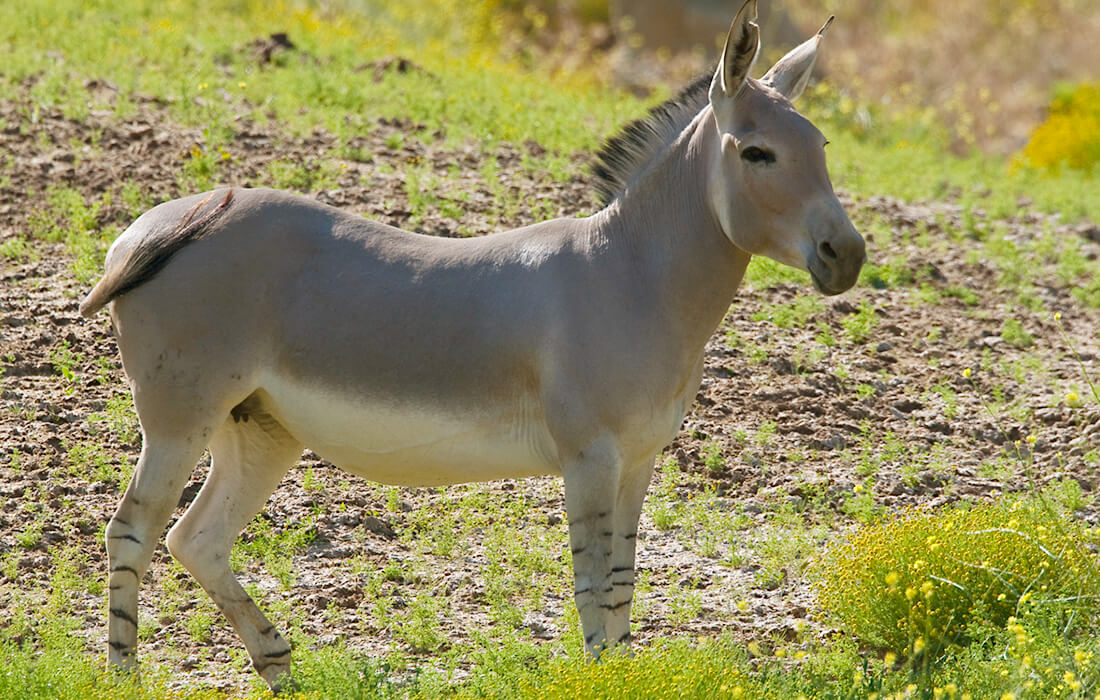This is an image of a unique animal that resembles a cross between a zebra and a donkey, possibly a rare zebra hybrid or mule with unique features. The animal is relatively small and is viewed from the side, with its head facing right and tail to the left. It has a dark grey, almost hairless coat, with a distinctive black and white mane. Its underbelly is white, contrasting with the solid grey of its body. The legs feature thin black stripes that go up to the knees. The animal has large ears that are black inside, black eyes, and a grey snout with visible nostrils and mouth. It's standing in a field under sunny conditions, with yellow and green brush, grasses, and small plants sprouting from the dirt. The background includes a mix of green leaves, some brown areas, and yellow flowers, possibly dandelions. The tail is dark and is captured in a flapping position towards its body.